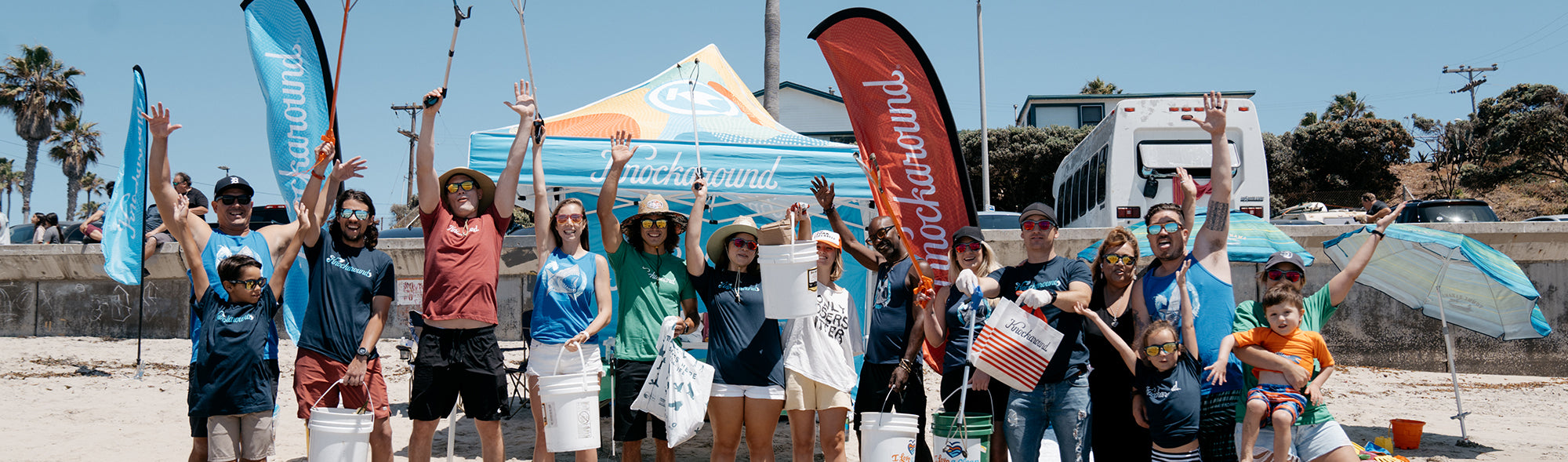A vibrant color photograph captures a long row of people waving their arms and cheering in front of a beach scene. The group, dressed in casual beach attire like shorts and t-shirts, holds white five-gallon buckets and bags, suggesting they might be participating in a beach cleanup or a communal event. The joyous crowd faces the camera with broad smiles, clearly enjoying their time by the sea. Behind them, a lively beach setup is visible, featuring several flags—red and light blue with white writing, possibly reading "knock around." These flags flutter in the breeze alongside beach umbrellas sticking out of the sand and an outdoor canopy tent bearing the same inscription. Sand, palm trees, and larger green trees further enhance the scenic backdrop. In the background, a white tour bus is parked, adding to the sense of a well-organized event. The sky, a light blue, completes this lively and celebratory beach scene.